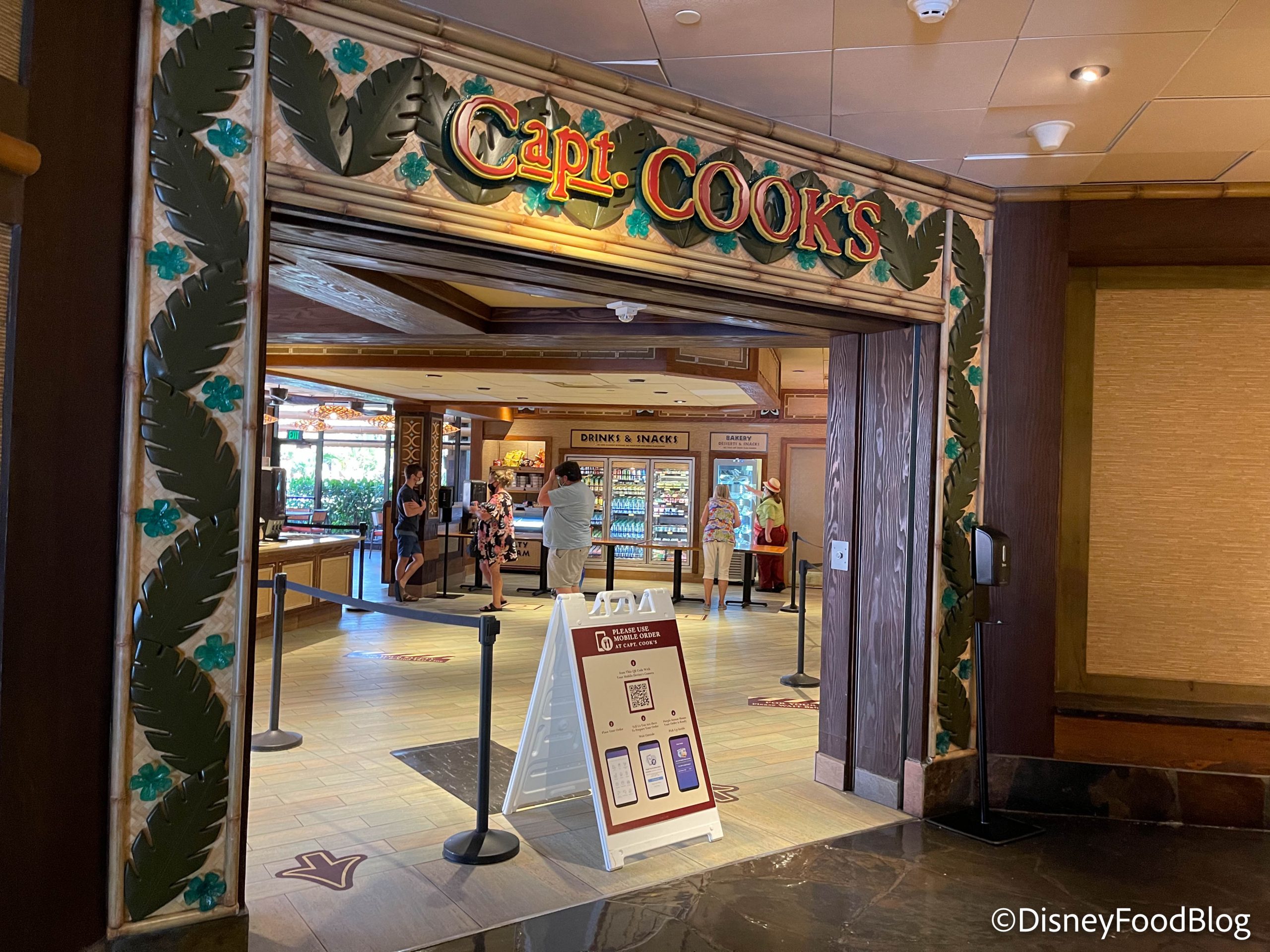The image showcases the entrance to a restaurant named Captain Cook's, possibly located within a mall. The entrance is adorned with decorative leaves around the sign bearing the restaurant's name in bold red letters. Standing before the doorway, a sign features an infographic with a QR code and phones. Inside, fridges labeled "drinks and snacks" as well as a bakery section can be seen against the wall. The restaurant is bustling with activity, with several people, some wearing masks, either standing around, talking, waiting in line, or examining the snack case. On the left side of the image, there is a visible counter and a window. The bottom right corner of the image contains text with a copyright symbol and the name “Disney Food Blog” in white. Additionally, arrows on the floor guide the movement of patrons within the establishment.